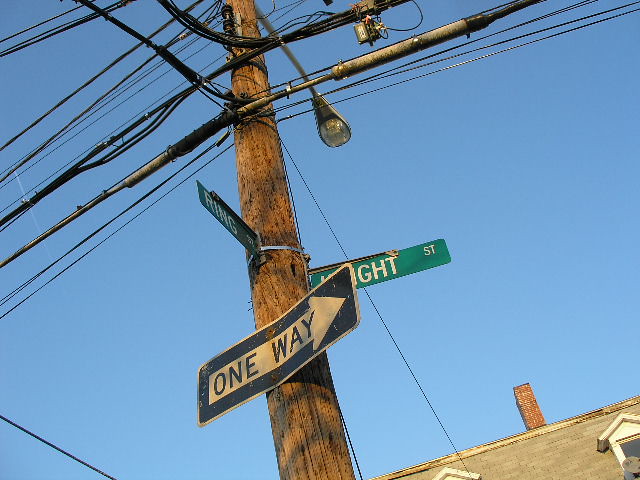In this outdoor photograph, we see a weathered wooden electrical pole showing signs of age through its dark brown, chocolate brown, and black streaks. The pole is festooned with numerous power lines in dark gray and black hues. At the top, there's a light-gray streetlight with a teardrop-shaped glass bulb. Affixed to the pole are three street signs: a dark blue "One Way" sign with white text and an arrow pointing to the right, a partially visible green sign with the letters "G-H-T-S-T" indicating "Night Street," and another green sign for "Ring Street" pointing straight. These signs are held in place with metal rings.

The background features a cyan blue sky and a building to the right side of the frame. The building has a prominent red brick chimney, gray shingled roof, and two overhangs near white windows—one partly cut off by the edge of the image. The overall scene captures the intersection setting beneath a clear sky, tying together the elements of urban infrastructure and residential architecture.